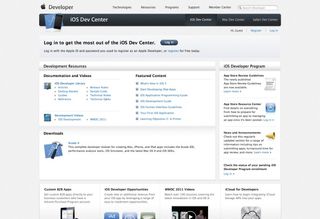The image shows a website with a low-resolution display, making the text difficult to read. On the left side, an Apple logo is visible alongside the word "developer." Towards the right, there are several navigation links, although the poor resolution prevents their content from being deciphered. Below this header section, a prominent black band features the text "iOS Developer Center" in white.

To the right of this banner, there are additional navigation elements, but these too are unreadable due to the low quality of the image. Following the black band, the background switches to white, displaying a blue button that is similarly illegible. Below the button, the page shows extensive textual content in blue and black fonts set against a primarily white or light gray backdrop. The readability of this text is severely compromised by the poor resolution; even the largest words are unclear.

The page employs a consistent color palette including white, gray, black, blue, and yellow. It appears well-organized with distinct sections separated by spaces and bullet points. Certain sections are labeled with bullet-point headings like "Featured," though the exact wording is indiscernible. Icons adorn the sides of these sections, suggesting a structured and thoughtfully designed layout, despite the image quality issues.